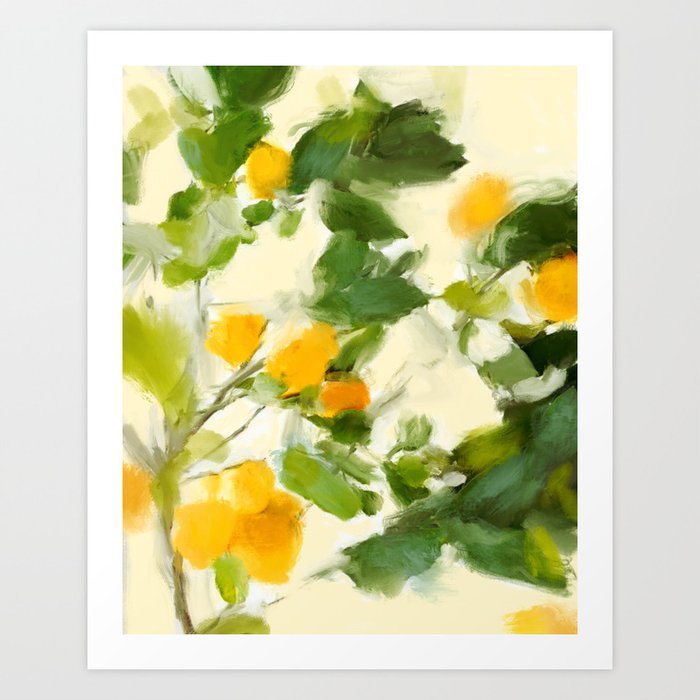The painting, displayed on a light grey or white wall, features a rectangular shape oriented vertically with a prominent white frame. The artwork itself is a delicate blend of various elements, including diverse patches of yellow and green, possibly representing abstract flowers and leaves. Dominating the scene are vibrant clusters of yellow flowers that bear a resemblance to lemons, suggested by their oval, lumpy shapes. These lemons and flowers are intertwined with bright, often shiny green leaves, creating an impressionistic visual feast. A grey, vertical branch adorned with green leaves punctuates the left side of the painting. The background is infused with soft light yellow hues, evoking a sense of 'La Dolce Vita' and reminiscent of serene Italian landscapes.